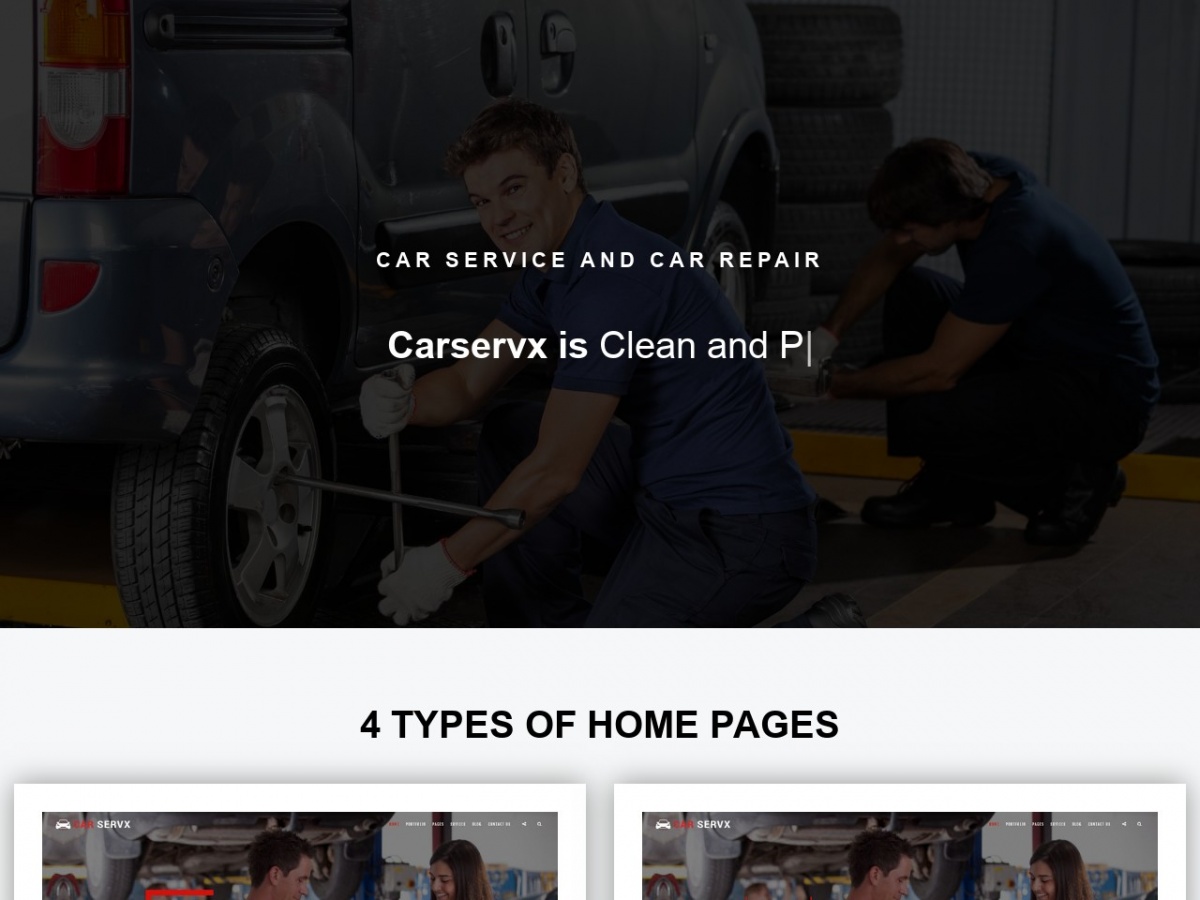This image is a screenshot taken from a person's computer screen, displaying a dark-themed webpage related to vehicle services. Centered prominently on the screen is the text "Car Service and Car Repair" written in clear white font. The background is predominantly dark, but faintly visible is a mid-action image of a mechanic. This mechanic is holding a lug wrench—a tool resembling a plus sign used for removing tire lug nuts. He is positioned towards the center of the image, smiling as he turns his head towards the camera. Behind him, a large vehicle with sizable wheels is partly visible. Another individual, whose head is bent down, appears to be working near the front of this vehicle.

Scrolling further down the screen, additional text in white reveals "CarsServX is clean and pee," with the cursor blinking nearby, indicating ongoing typing or editing. Additional webpage features are noted at the bottom, mentioning "Four types of homepages." However, only two clickable options are visible while the rest are cut off due to the limitations of the screenshot size.